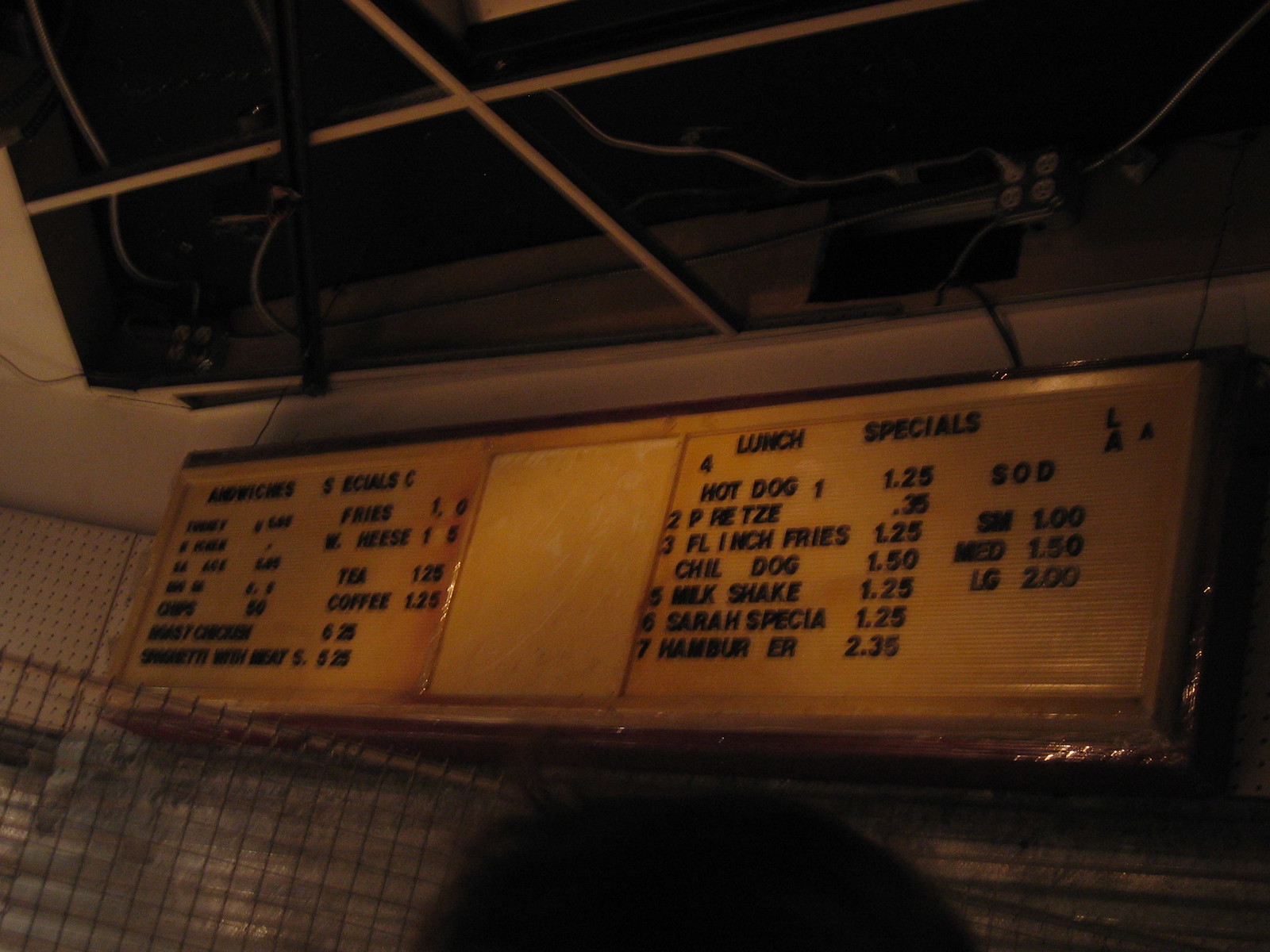The image captures a cropped view of a vintage-style restaurant menu, with a clear look at the ceiling and parts of the tiled walls in the background. The ceiling features white metal square panels interspersed with black or reflective material, possibly a venting system or a space where tiles should be, exposing some wires, suggesting the view might be up into the ceiling.

The tiled wall in the background showcases a mixture of very small white tiles, which might be pegboard, at the top left, transitioning to slightly larger bluish-gray square tiles that cover the entire wall area beneath the menu sign.

The rectangular menu sign itself appears aged and discolored to a yellowish hue, with black lettering displaying various menu items. A less discolored square in the middle hints at an area once containing text or imagery, now faded or removed. On the left side of the sign, there's an indistinct menu item, blurred, but the price for coffee is visible at $1.25.

To the right, black stick-on letters spell out "Lunch Specials" with items such as hot dogs, pretzels, french fries, chili dogs, milkshakes, and hamburgers advertised. Some letters are missing, but visible prices range from $1.25 to $2.35. Further to the right, drink prices are listed for small, medium, and large sizes at $1, $1.50, and possibly $2 respectively. The overall ambiance suggests a nostalgic snapshot of a simpler dining era.